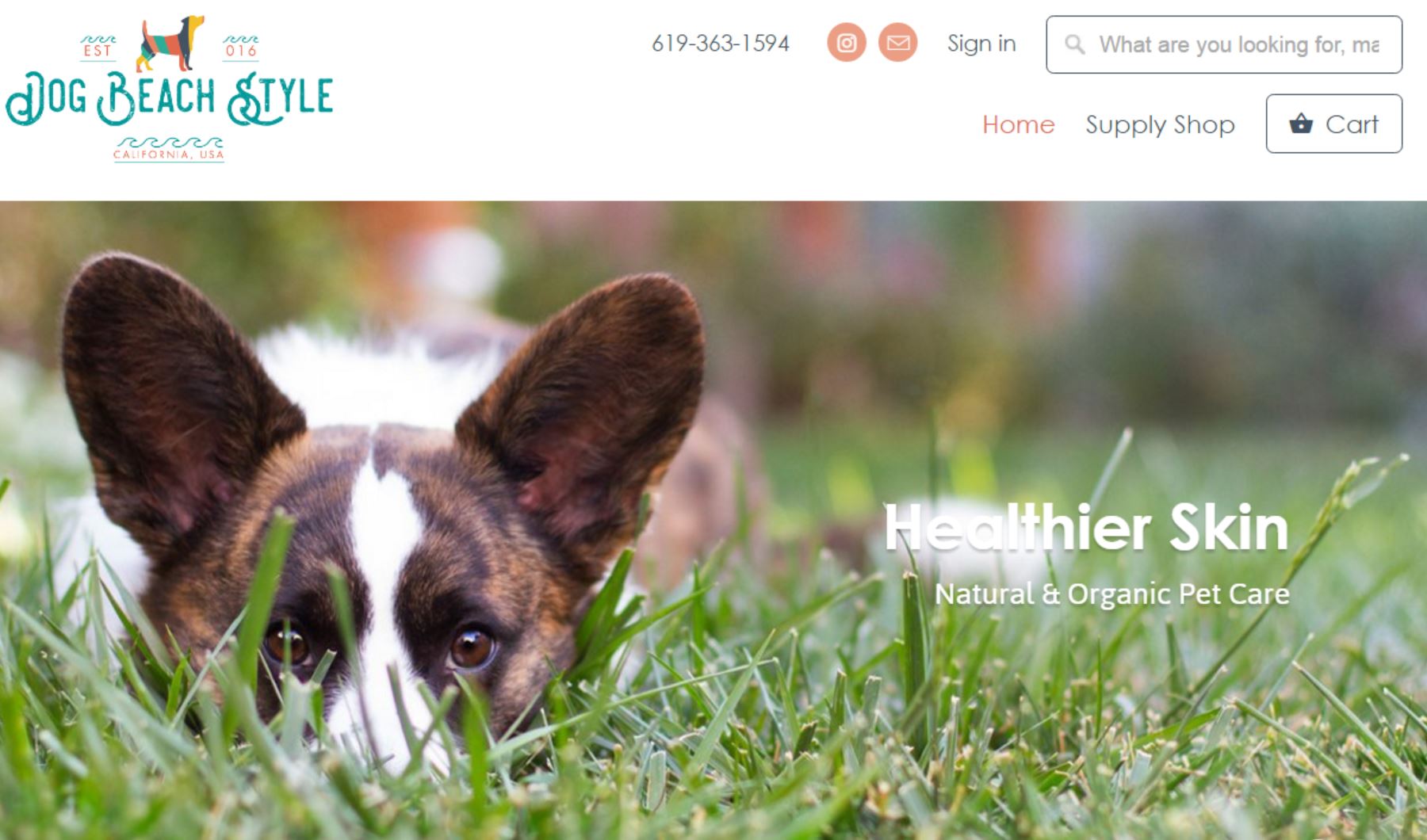This image showcases a vibrant and welcoming website dedicated to dogs. Prominently featured in the top left corner is the site's name, "Dog Beach Style," rendered in blue text with an accompanying colorful rainbow dog icon above it. Surrounding this are various labels, enhancing the site’s navigational clarity. Adjacent to this on the right, there is a prominently displayed contact number in black, flanked by two red circles. Further right, users will find a black sign-in option and a black rectangle containing a search bar labeled, "What are you looking for, MA?" 

Beneath this navigation bar, a red home icon is visible, followed by links to the "Supply Shop" and "Cart," both outlined in black. The main body of the page features a captivating image of a dog's face nestled in the grass. The dog’s eyes and ears are in clear focus, revealing deep brown eyes set above a white patch of fur between them, contrasting with the primarily brown fur of the face. The dog's body, visible in the background, continues this mix of brown and white fur.

On the right-hand side of this section, text reads, "Healthier Skin, Natural and Organic Pet Care," emphasizing the site's dedication to pet wellness. The entire background of the image is composed of lush green grass, with the foreground sharply in focus, while the background grasses are artistically blurred. Various color hints, including black, green, red, and traces of purple, subtly mix within the blurred background, adding depth and visual interest to the scene.